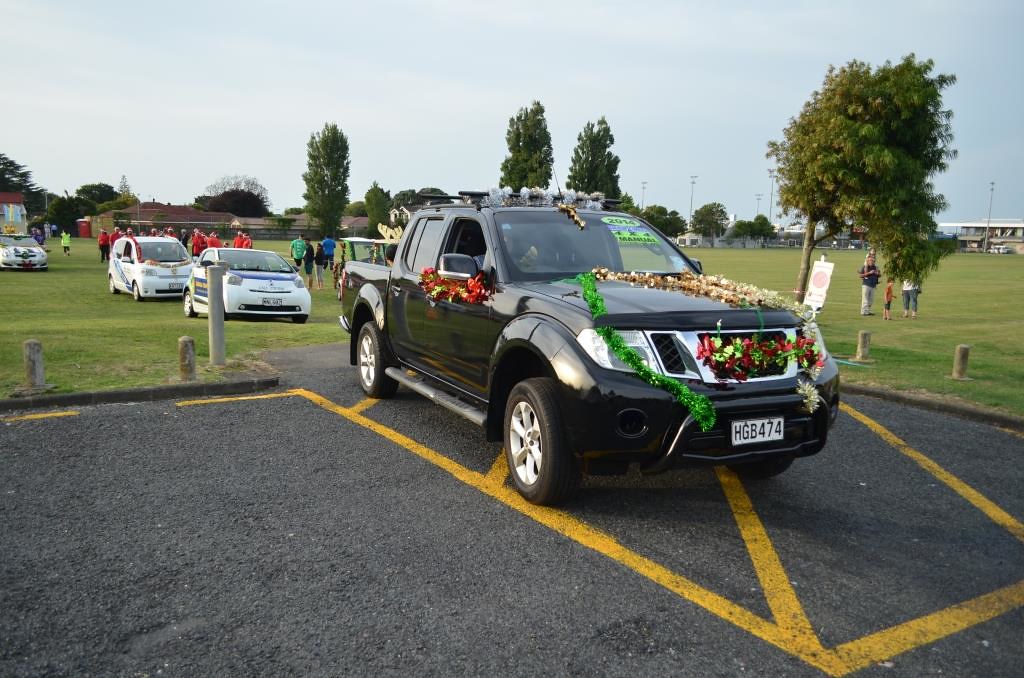The image depicts a lively outdoor scene at what appears to be a car show held in a spacious parking lot. Central to the photograph is a black pickup truck adorned with floral wreaths and garlands, and the license plate reads HGB 474. The truck is prominently positioned within yellow painted lines, indicating a designated parking space. To the left and rear of the black truck, on a grassy area, three white cars are lined up. Surrounding the vehicles, a diverse group of people clad in brightly colored shirts—including red, green, blue, and more—can be seen mingling. In the background, there are trees, a fence, some buildings, and a tall or possibly two-level building to the far right. The sky is predominantly blue with scattered clouds, adding to the overall vibrant and festive atmosphere of the event.